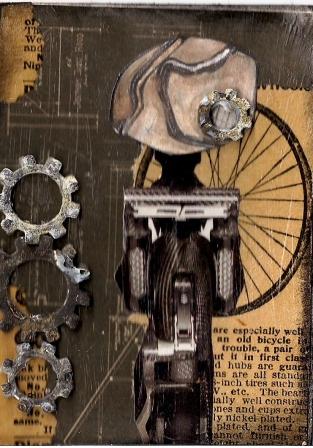The artwork features a detailed and intricate assembly of various small objects forming a larger, cohesive image, set against a scratchy brown wooden background. On the left side near the bottom, three interlinked metal cogs add a mechanical element to the piece: the top cog is silver, the middle cog is brown and rusty, and the bottom cog is silver but slightly rustier than the top one. At the center of the composition, assorted pieces of scrap creatively depict the back of a woman wearing a dress and a large pink bonnet. In front of her, a wheel lies on a scrap of yellowed newspaper with fragmented black text that reads, "Well, an old bicycle trouble a pair, if in first class. Hubs are guards, are all standard 8-inch tires such," though the text is partially obscured and incomplete. Overall, the majority of the image is in brown hues, enhancing the rustic and vintage atmosphere of the artwork.